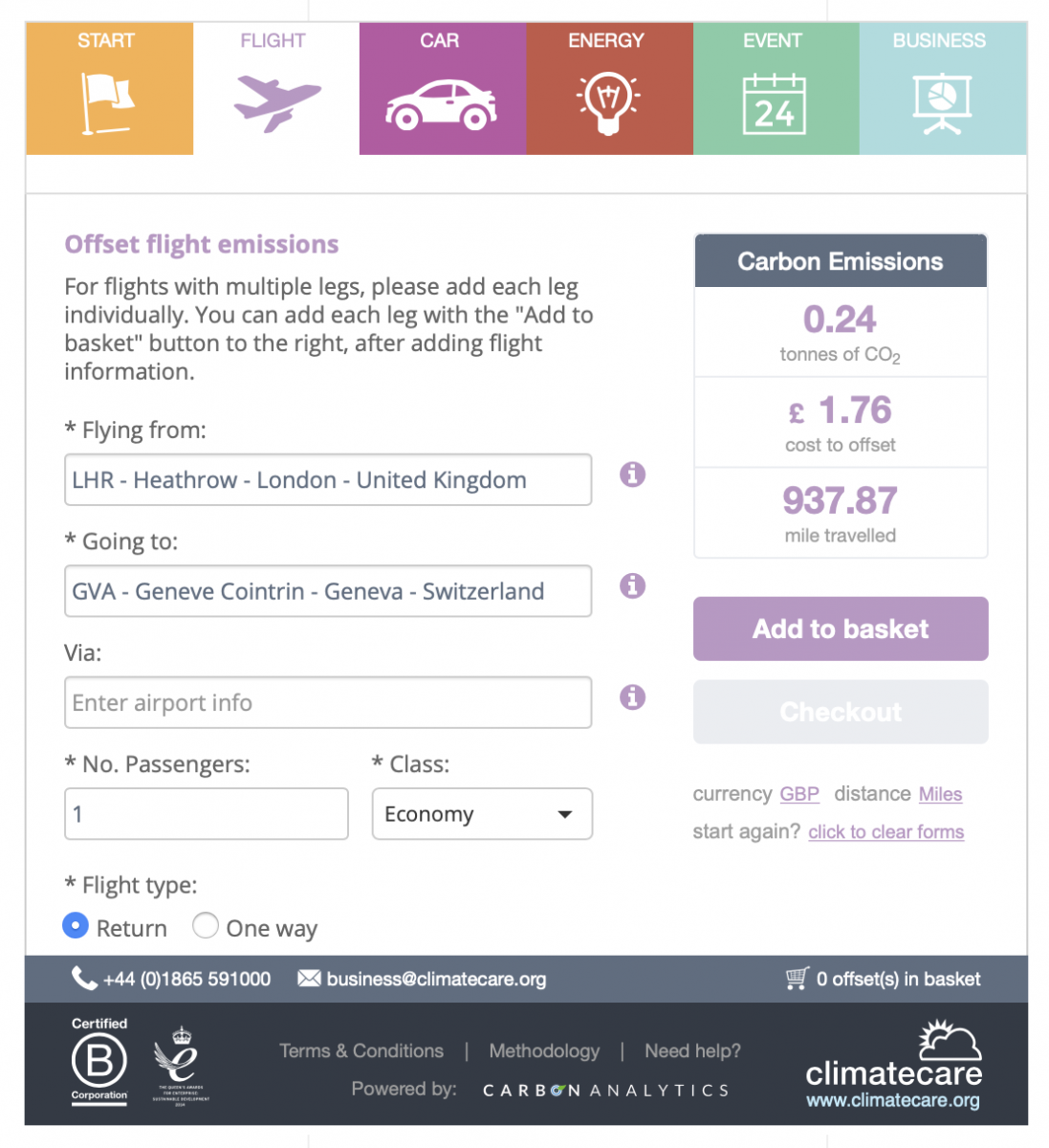**Detailed Caption for Webpage Image:**

The webpage displays a user-friendly interface with multiple colored buttons, each representing different functions and categories through text and silhouettes:

1. **Orange Button**: Located on the left-hand side, it features the word "Start" in white at the top center, accompanied by a white flag and pole icon to the right.
2. **White Button**: This square button displays a purple airplane and the word "Flight" in the center.
3. **Purple Button**: Featuring a car silhouette facing left, the word "Car" is centered within this square.
4. **Brown Button**: Reads "Energy" with a lightbulb at the lower center, emitting dashes of light illustrated by white lines.
5. **Teal Button**: Labeled "Event," depicting a calendar with the number "24" at the bottom.
6. **Green Button**: Named "Business," it shows a projector screen with a pie chart.

Below these are functional sections within a white rectangle bordered by a thin black line:

1. **Flight Emissions**: Mentioned as "Offset Flight Emissions" in purple text.
2. **Flight Information Instructions**: Black text guides users on adding multiple flight legs individually using an "Add to Basket" button to the right.
3. **Flight Details**:
   - Flying From: Rectangular box labeled "LHR-Heathrow-London-United Kingdom."
   - Going To: Another box labeled "GVA-Geneva-Cointrin-Geneva-Switzerland."
   - Via: Line followed by a gray rectangle for entering airport information.
4. **Passenger and Class Selection**:
   - No. of Passengers: White rectangle showing "1."
   - Class: Drop-down box selected as "Economy."
5. **Flight Type**: Includes radio buttons for "One Way" (white, unselected) and "Return" (blue, selected with a white dot).

Additional contact information and features are displayed:

1. **Contact Details**: 
   - Telephone: +44 (0)1865 591000
   - Email: business@climatecare.org
   - Shopping Cart: Indicates "0 offsets(s) in basket."
2. **Certifications and Logos**:
   - B Certified Corporation
   - E-logo with a crown and wings.
3. **Company Branding**:  
   - Climate Care logo with a cloud and sun, website URL: www.climatecare.org (in cyan blue).
   - Centered text includes "Terms and Conditions," "Methodology," and "Need Help?" separated by gray lines.
   - Footer reads "Powered by Carbon Analytics" with "Carbon" in bold white and "Analytics" in gray.

This detailed layout ensures clear navigation and access to essential information for users planning their trips and managing flight emissions.